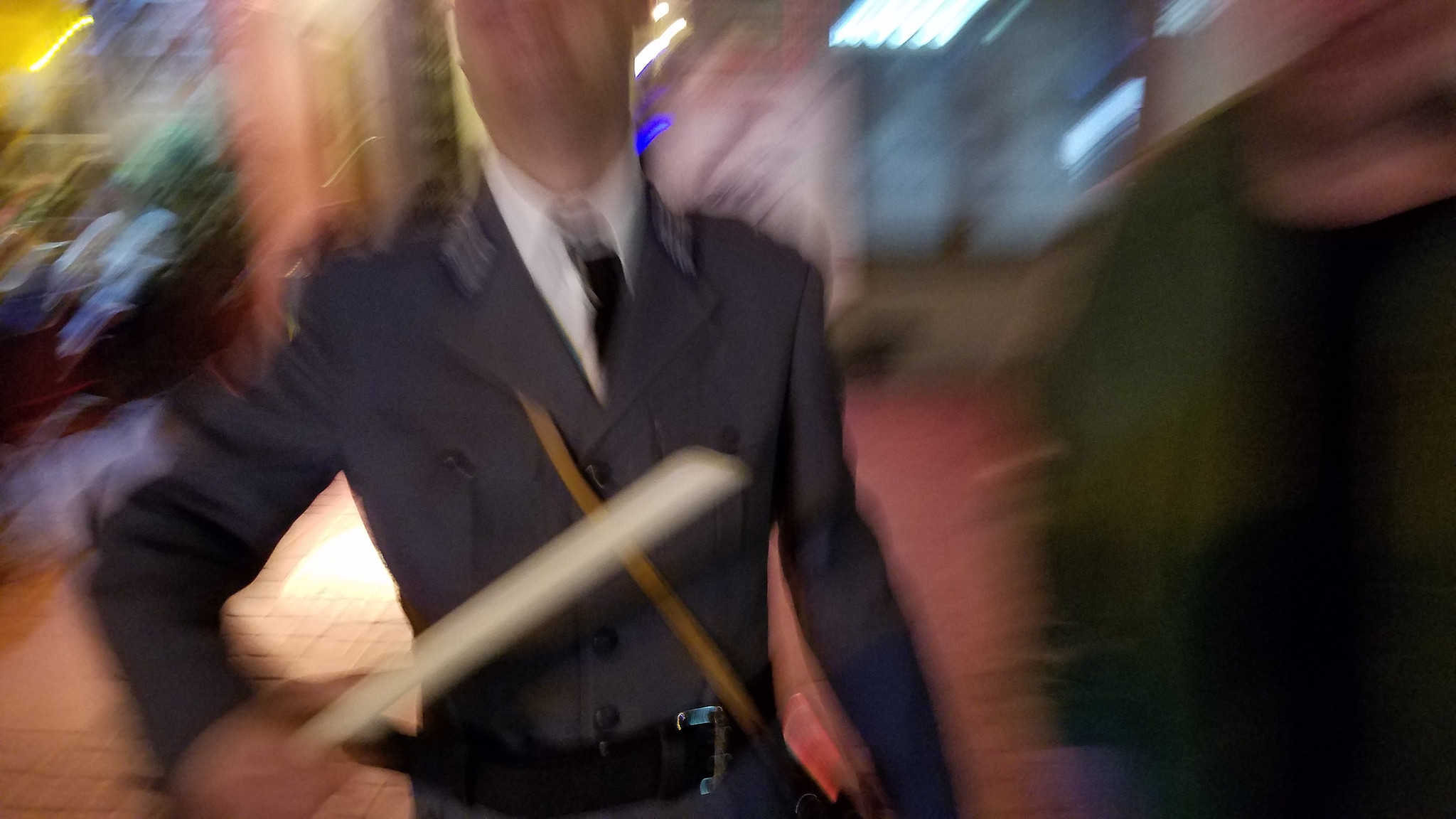The image is blurry due to camera motion, with a noticeable blur from the upper right to the bottom left. The focus is on two Caucasian males. The person on the left is wearing a bluish-gray uniform, which includes a white button-up shirt and a black tie, all buttoned up. He has a black leather belt and a brown strap diagonally across his body, possibly from a messenger bag. In his right hand, he holds a long, cylindrical white object, possibly a rolled-up paper or a baton. The second person, on his right, wears a black shirt with a green jacket or coat over it. The background suggests an indoor setting, potentially a building, with visible windows and fluorescent lights. There's an older woman seated in the background. To the left side of the image, there's an entryway to another room and some greenery in the far left corner. The floor appears to be an off-red or maroon color.